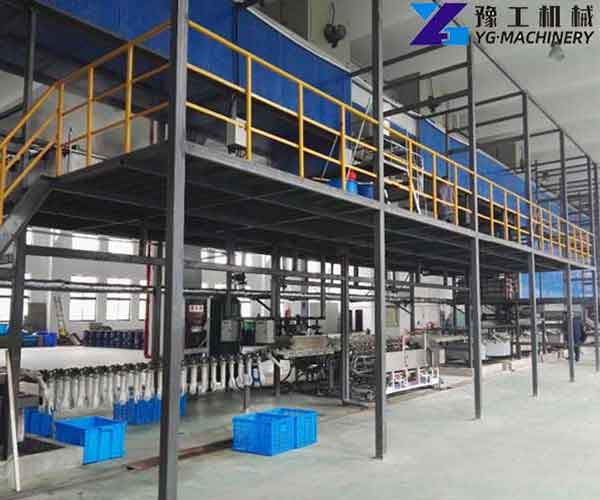The image depicts the interior of a factory, likely sourced from a manual or report. Prominently featured in the top right corner are four possibly Chinese or Japanese characters, accompanied by a logo resembling an X, with one line purple and the other blue, alongside the text "YG-MACHINERY" in black. The factory itself appears on two split levels. The ground level is concrete, and steel bars support a second story with a yellow guardrail running along its perimeter. The roof of the second floor is accented with blue. The ground floor is dotted with machinery and blue containers, and seems to be involved in the production of medical gloves, evidenced by numerous hand-shaped mannequins being dipped into a substance, likely silicone. Sunlight streams through windows on the left side, illuminating the gray walkways and the gray poles supporting the upper platform. A yellow staircase provides access to the second story, and a figure can be seen in the far right background of the image.